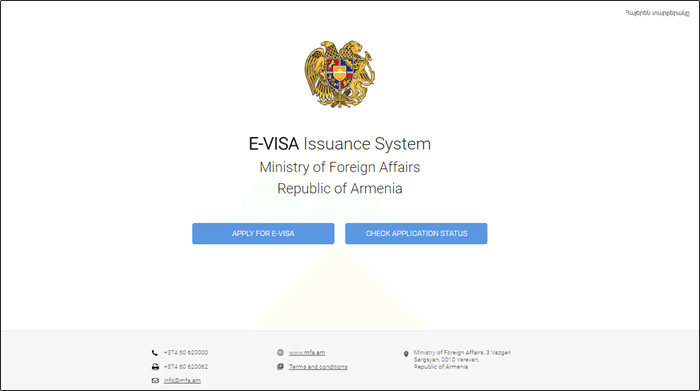The image is a screenshot of a webpage with a clean, white background. Dominating the center of the page are two gilded figures; on the left, a stylized logo that resembles either an eagle or a lion or leopard, and on the right, a crest featuring a red and blue shield—red on the upper part and blue on the lower. The text "E-Visa" is prominently displayed in bold black font, emphasizing the service. Beneath this, "INSURANCE SYSTEM" is written with capitalization of the initial letters "I" and "S."

Below the main heading, there is a line of smaller text: "Ministry of Foreign Affairs," with the key letters "M," "F," and "A" capitalized. Following this is another line stating "Republic of Armenia," with "R" and "A" similarly capitalized. 

In the top right corner of the webpage, there is text in what appears to be Russian. Towards the lower section of the page, there are two prominent blue buttons with white text. The button on the left reads "Apply for E-Visa," and the one on the right reads "Check Application Status."

At the bottom of the page, contact information is provided:
- A telephone symbol paired with the number +374-60-620-0000
- A fax symbol alongside the number +374-60-620-062
- An email icon followed by the address info@mfa.am
- A website link www.mfa.am

Additionally, there are icons for documents, one labeled "Terms and Conditions" with an underline, suggesting it is a clickable link.

The footer also contains address details located in a mid-gray rectangle, reading: "Ministry of Foreign Affairs, 3 Vazgen Sargsyan, 0010 Yerevan, Republic of Armenia."